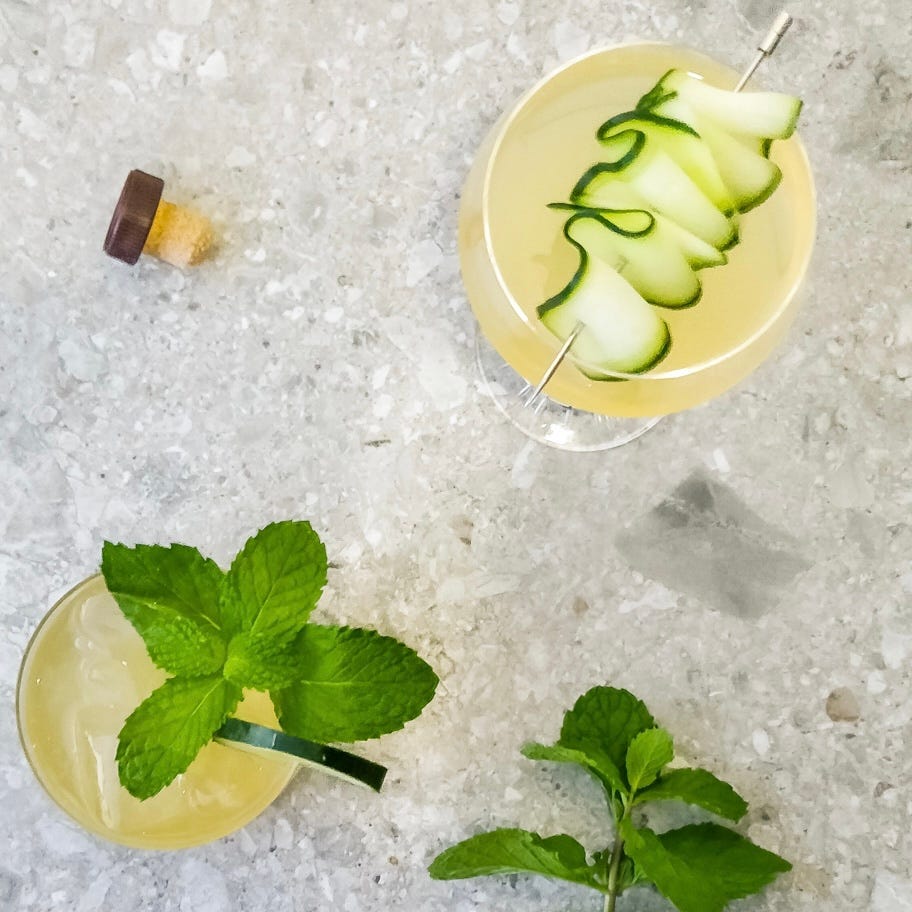The image depicts a top-down view of a marble countertop with a speckled pattern in tans and off-whites. In the lower left corner, there is a glass containing yellow liquid with ice cubes, mint leaves floating on top, and a cucumber slice on the rim. The upper left corner features a wooden cork with a round brown cap. The lower right corner also has mint leaves scattered about, while the upper right corner showcases a glass with light yellow liquid. This glass is adorned with a long cucumber slice, cut into a wavy pattern and skewered on a metal toothpick that rests across the top of the glass. The differing shades of yellow in the drinks and the distinct glass designs suggest they might be variations of the same cocktail.